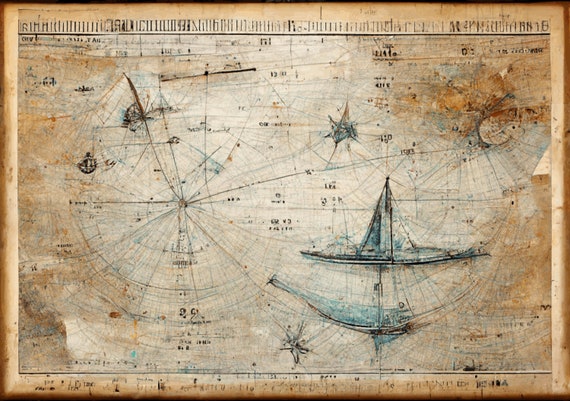The image depicts a very old and worn paper map, with a predominant beige and brown coloration, indicative of age. The map features numerous connected lines and grid patterns that intertwine across the entire surface. In the bottom right corner, there's a small blue ship, partially obscured by what appears to be a faint shadow of another similar illustration. The top right hosts a small orange or brown structure, intricately linked by lines to other ships mostly on the right side of the map, while smaller ships on the left connect to various central points. The map’s edges are darkly aged, suggesting extensive exposure and wear. The center features coordinates that are difficult to decipher. Splashes of blue ink are scattered throughout, adding a distinctive color contrast against the backdrop of lighter tan to dark brown shades. There are also several vertical lines stretching across the top, possibly indicating a measurement system or latitude references, yet no specific land structures are visible, enhancing a sense of mystery and fantasy.